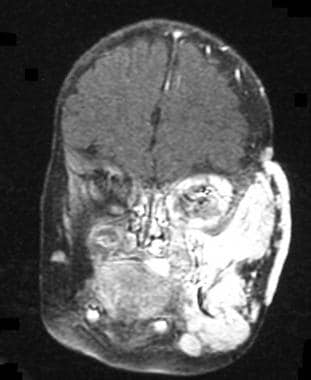The image is a detailed black-and-white cross-section, likely from a CAT scan or MRI, depicting a human skull set against a consistent black background. The central head is displayed in tones of black, gray, and white, giving it a slightly holographic and 3D appearance. The skull’s structure is clearly defined, with bright white eye sockets, especially the right one standing out more distinctly than the left. The brain is visible and shaded in light brown or gray tones. There are no visible teeth and no text, animals, buildings, or mechanical objects in the image; the focus remains solely on the intricate details of the skull and brain within the dark background.